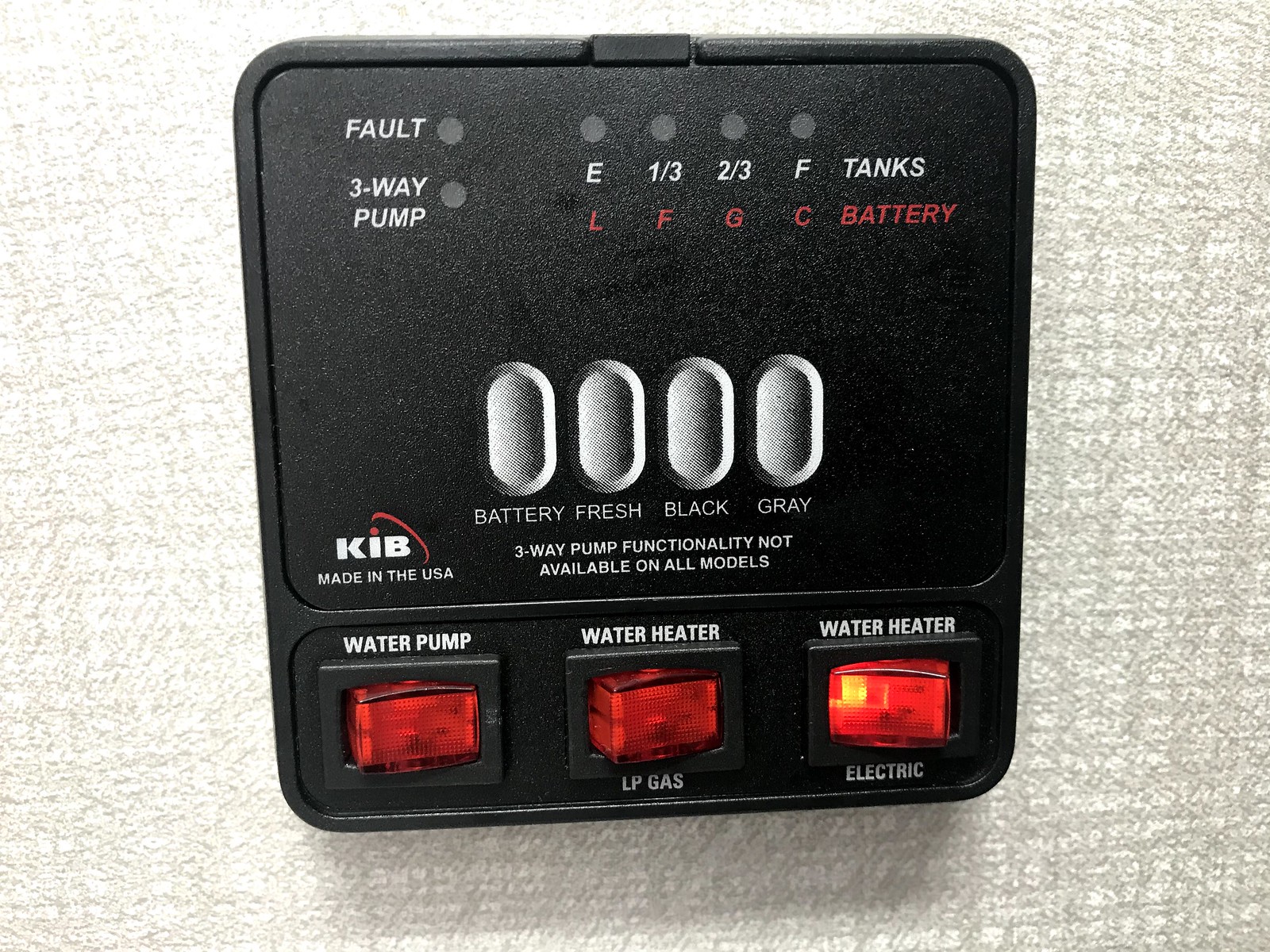This photograph captures a close-up view of a wall-mounted control panel, predominantly black, featuring a series of switches, lights, and informational text. The panel consists of three red toggle switches at the bottom: the left switch labeled "Water Pump," the middle switch labeled "Water Heater" (with "LP Gas" below it), and the right switch labeled "Water Heater" (with "Electric" below it), which is flipped and lit up. Above the switches, there are two rows of indicator lights with labels. The top row includes "Fault," "Three-Way Pump," "E," "1/3," "2/3," "F," "Tanks," while the bottom row includes "L," "F," "G," "C," and "Battery." None of these lights are currently lit. Further up the panel are four silver oval buttons marked "Battery," "Fresh," "Black," and "Gray." The text "Three-Way Pump functionality not available on all models," positioned at the lower part of the panel, provides additional detail. To the left, a logo reads "KIB Made in the USA," accompanied by an arc design. The background behind the control panel is a textured tan color, enhancing the panel's visibility and detail.